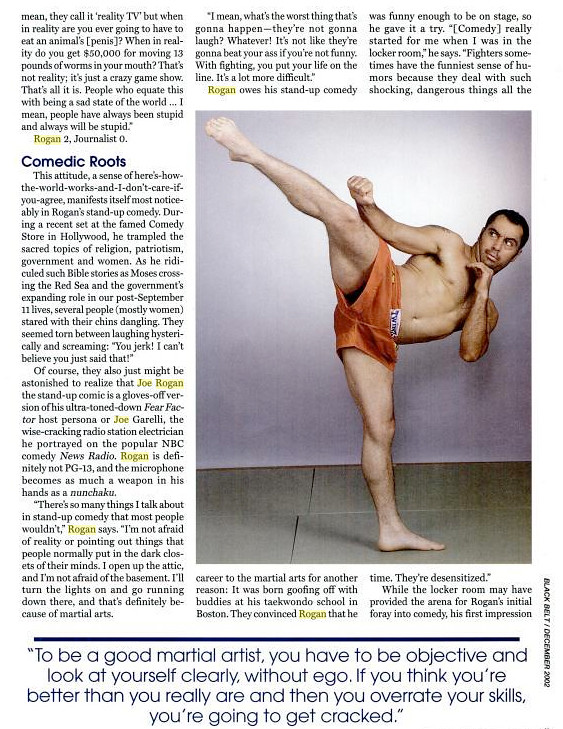The image depicts a shirtless man, likely in boxing trunks, barefoot on a white tiled floor. He strikes a dynamic kickboxing stance, standing on his left foot with his right leg extended high in the air, his body leaning to the left. His left arm is positioned under his chin while his right arm is raised with a clenched fist. The man's gaze is fixed upward towards his extended leg. He has short, dark hair and stands against a white background. Adjacent to him is a vertically oriented black-and-white news article with yellow highlights on the words "Comedic Roots," "Rogan," and "Joe." At the bottom of the article, a prominent quote reads, "To be good at martial arts, you have to be objective and look at yourself clearly without ego. If you think you're better than you really are, and then you overrate your skills, you're going to get cracked." The overall composition is a detailed blend of imagery and text, suggestive of a publication or feature article.